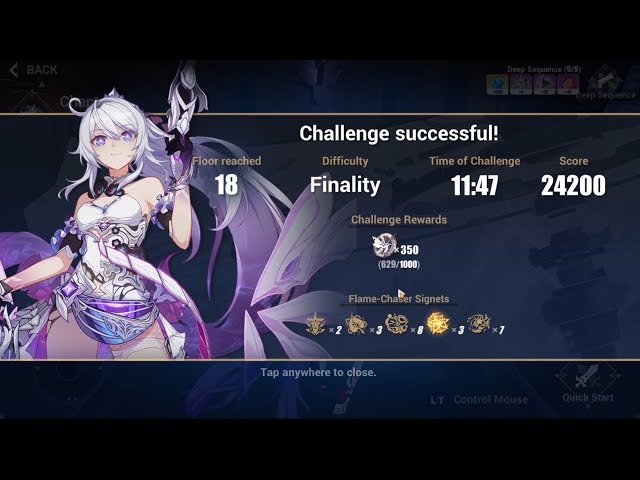The image appears to be a screenshot from a video game showing the results screen of a completed challenge. Dominating the left side of the screen is a character—an attractive anime-style young woman with long, whitish-blonde hair and striking purple eyes. She is dressed in a sci-fantasy outfit, featuring a very short dress that is long in the back, and holds what seems to be a ray gun in her left hand. She is also wearing purple mittens or gloves.

The background is partially blacked out, emphasizing the results overlay. The text "Challenge Successful" is prominently displayed in a light beige color at the top of a band across the screen. Key game stats are listed beneath: "Floor Reached: 18, Difficulty: Finality, Time of Challenge: 11 minutes 47 seconds, Score: 24,200." Additionally, the screen notes that the player has earned "350 Challenge Rewards" symbolized by gold coins and possibly signets displayed at the bottom. The image’s intricate details and fantastical elements suggest a high-energy, visually engaging game environment.